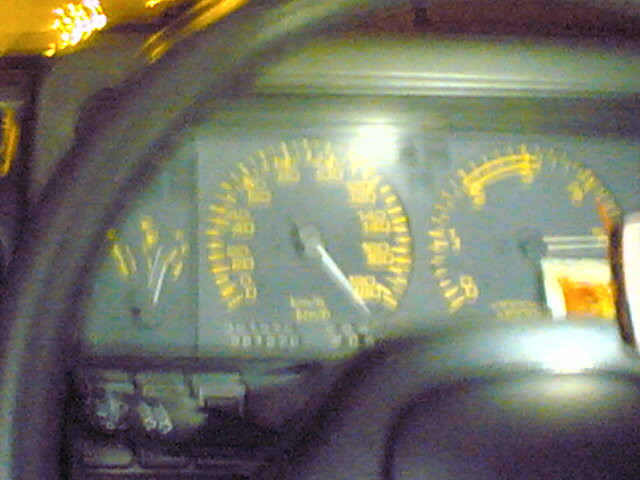This low-light, blurry photograph captures the dashboard of an older car, viewed through the space between the top-left and center portions of the steering wheel. The dashboard features manual dials, indicative of a vintage vehicle. Prominently visible are the speedometer, odometer, and fuel gauge, all set against a black background with yellow numerals and thin, white hands. In the top left corner, there's a reflection or external light source, adding a faint glow to the scene. Positioned against the right side of the odometer is a flat, square object with a white trim and a golden-orange center, possibly a piece of paper or a small card.